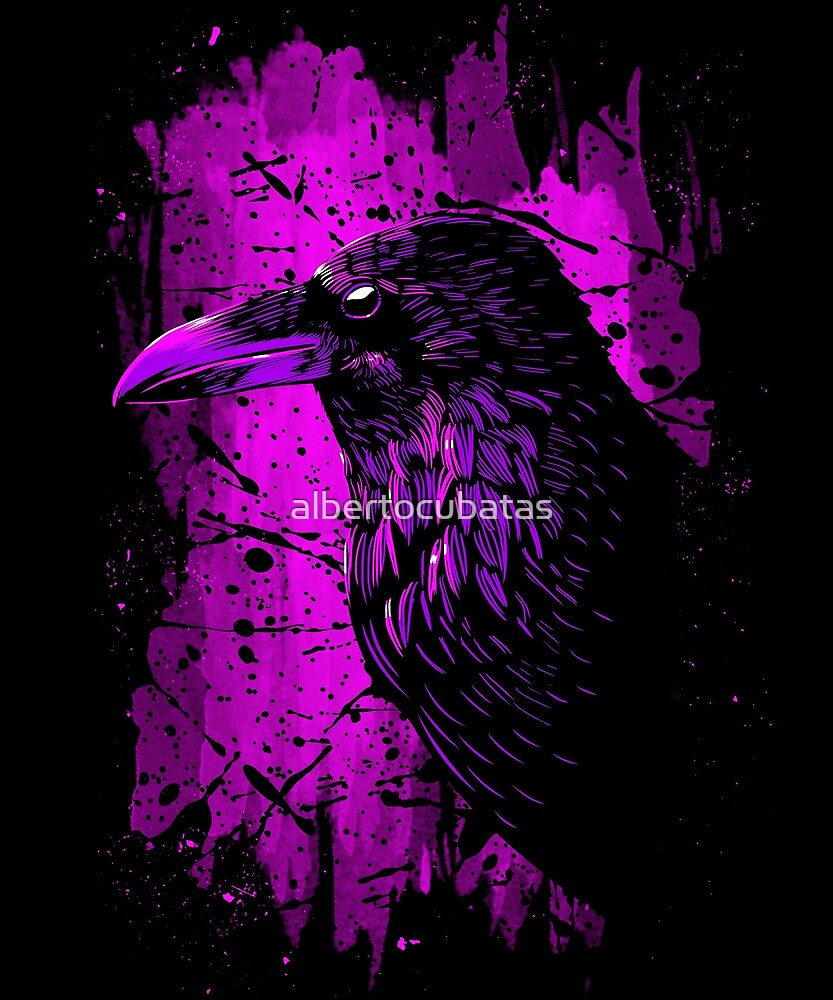This digital artwork features a striking, large raven positioned off to the right of the image. The raven is rendered in a combination of black, purple, and subtle pink shades, highlighting its prominent beak and attentive left eye, which is predominantly black with a white crescent at the top. The background is a dark, almost inky black with dynamic splatters and blotches of black paint dispersed across a vibrant, purple canvas that lies behind the bird. The composition's bold color palette includes hues of black, purple, pink, white, and gray, with particular attention to purple splashes in the middle. Text at the center reads 'Alberto Cubittus' lending a sense of mystery to the piece. The overall impression is one of fierce elegance, with the meticulously detailed raven and the chaotic beauty of the background converging to form a captivating visual experience.